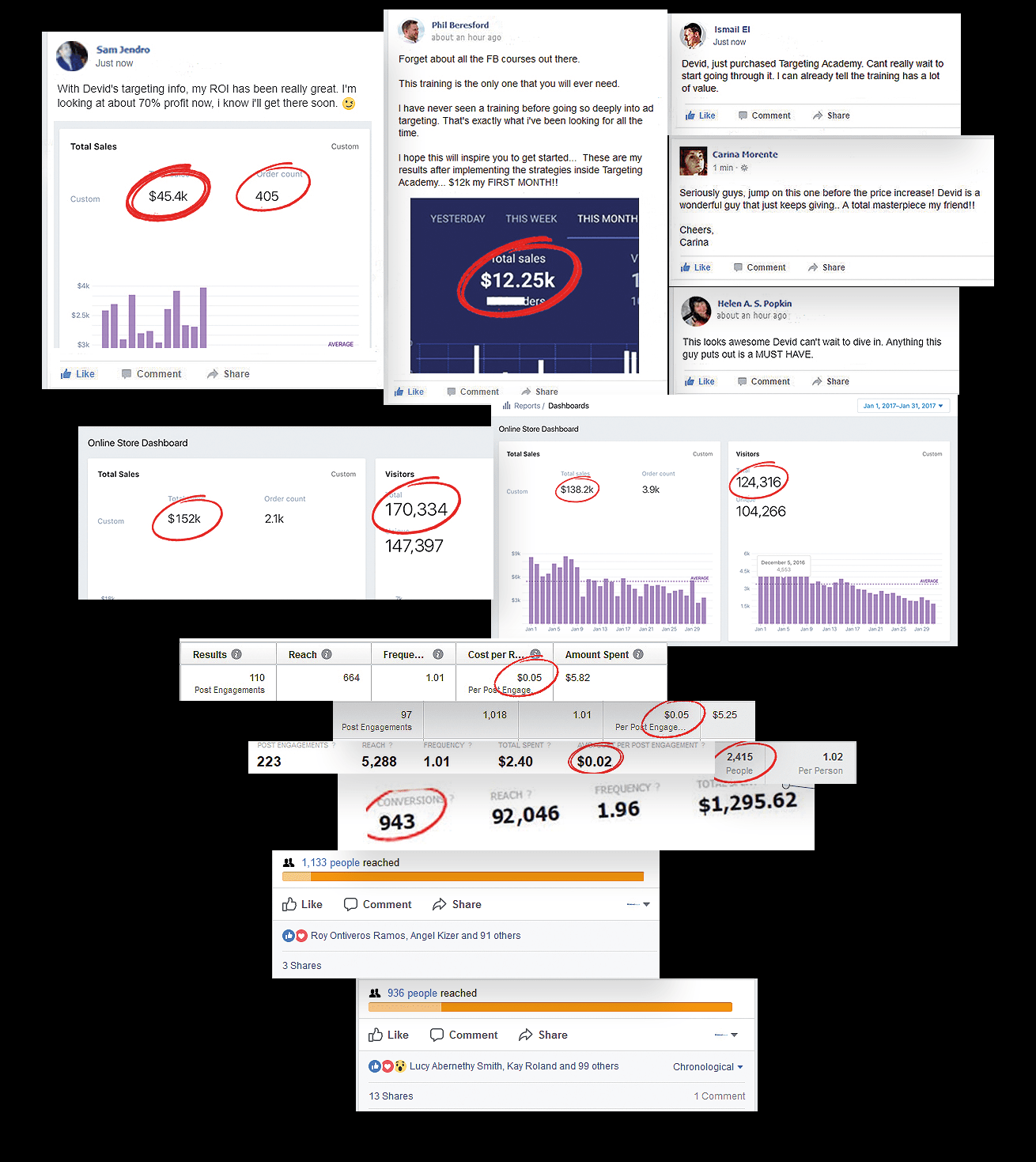This is a highly detailed image of a financial data screen, centered around various stocks, bonds, and informational quotes. The background is predominantly black, contrasting sharply with numerous white and rectangular elements of different shapes and sizes. Some rectangles are long and skinny, while others are taller and less wide.

Scattered across the screen are numbers and data points, some of which are circled in red marker, indicating areas of particular interest or importance. Towards the top, there are profile pictures along with messages. One notable message reads, "David, I just purchased Targeting Academy. I can't wait to start going through it. I can already tell the training has a lot of value."

At the bottom of the image, interactive elements such as likes, comments, and shares are displayed. An orange bar runs along this bottom section, visually segmenting the lower part of the screen. The overall aesthetic combines detailed financial data with user interactions, framed in a visually striking black and white contrast punctuated by red and orange highlights.